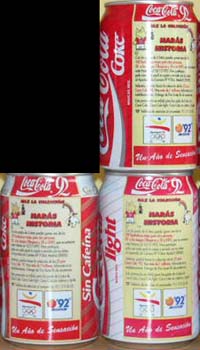The image is a composite photograph divided into four sections. The upper left section features a solid black box, creating a stark contrast to the other sections. The remaining three sections each display different views of a vintage Coca-Cola can. This retro can is characterized by its predominantly red and tan coloration, evoking a sense of nostalgia. Splotches of white lettering spell out the iconic Coca-Cola name multiple times across the various panels of the can. Additional red text is situated against the tan background, although the resolution and scale of the images make it difficult to discern this smaller print. The can also features smaller logos and labels adding to its vintage charm, but these elements remain largely unreadable. The overall arrangement provides a thorough visual exploration of the aged soda can, highlighting its historical branding and design elements.